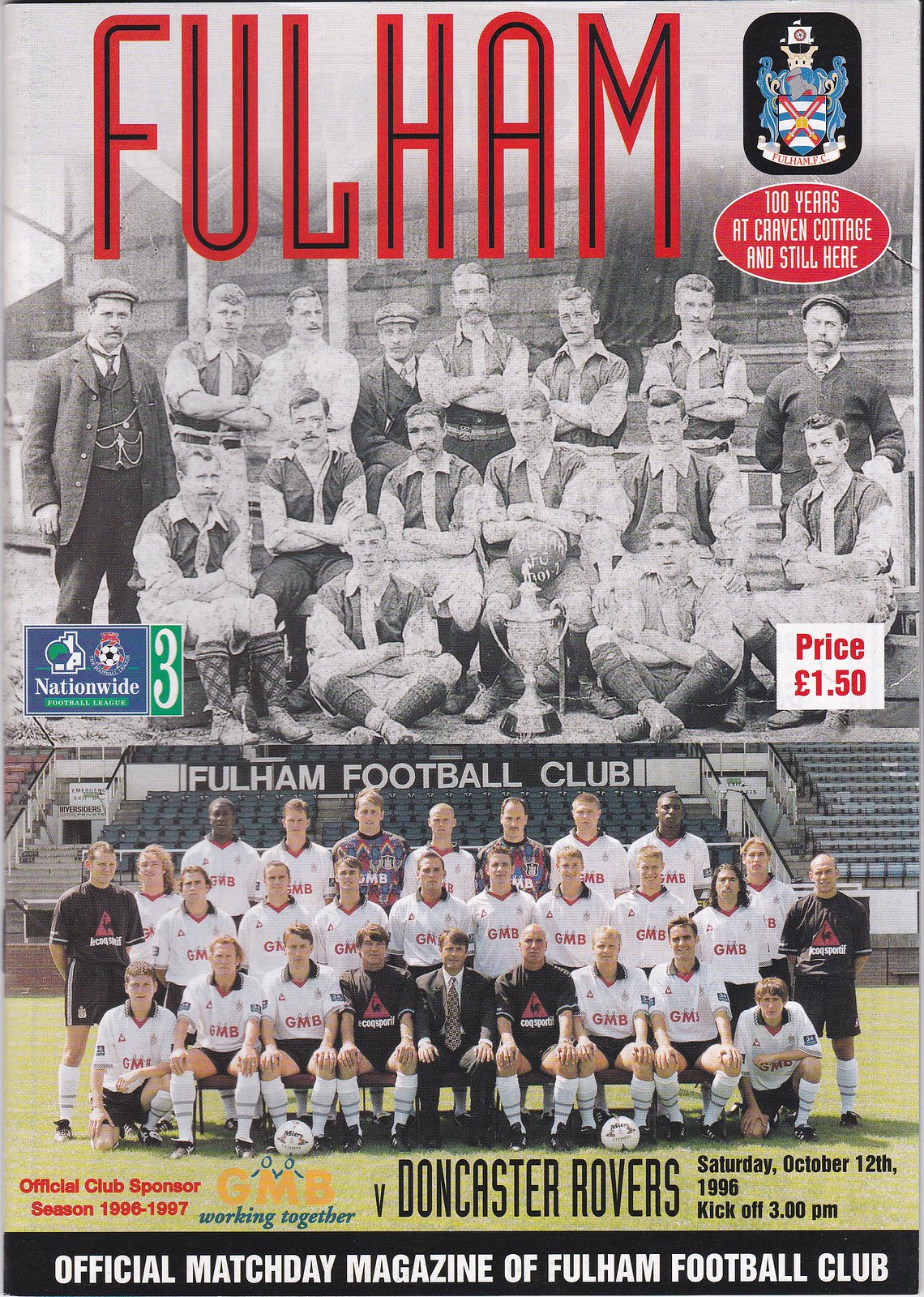This image appears to be the cover of an official match day magazine for Fulham Football Club. At the top, in bold red capital letters with black-filled centers, it prominently displays "FULHAM", occupying around the top 20% of the cover. To the right of the title, there's the club's crest and a red bubble with white text that reads "100 years at Craven Cottage and still here."

Below this, the cover is split into two halves. The top half features a black and white photograph of an old Fulham team, likely from the 1940s or 50s, with players displaying classic mustaches and hairstyles indicative of that era. The team is arranged in three rows: the front row sitting cross-legged on the ground, the middle row seated on chairs, and the back row standing. On the bottom left of this black and white section, the word "Nationwide" appears, and on the bottom right, a white box with red text displays "Price 150."

The bottom half of the cover presents a modern color photograph of the Fulham Football Club team, dressed in white shirts with red writing and black shorts. They are situated on the field with soccer balls in front, and the stands and bleachers visible in the background. Below this image, text details the official match information: "Official Club Sponsor, Season 1996-97, GMB working together vs Doncaster Rovers, Saturday, October 12, 1996, kickoff 3 p.m." At the very bottom, in a black box with white text, it reads "Official Match Day Magazine of Fulham Football Club."